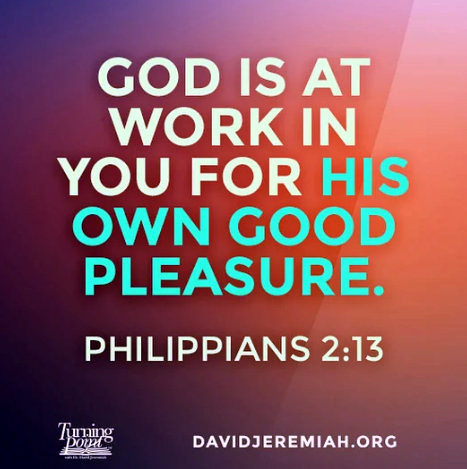This image appears to be a meme or advertisement promoting a religious message, likely intended for sharing on social media platforms such as Facebook. The background features a gradient starting with purple and blue hues in the top left corner, transitioning to lighter shades of red and pink. The central text is a biblical quote: "God is at work in you for His own good pleasure," with "His own good pleasure" highlighted in blue text while the rest of the text is in white. Below the verse, "Philippians 2:13" is written in a smaller, non-bold white font. On the left side of the image is the text "davidjeremiah.org," indicating a website, and in the bottom left corner, there is a "Turning Point" logo, which appears to be an open book. This image serves as a religious quote, likely associated with the teachings of David Jeremiah.